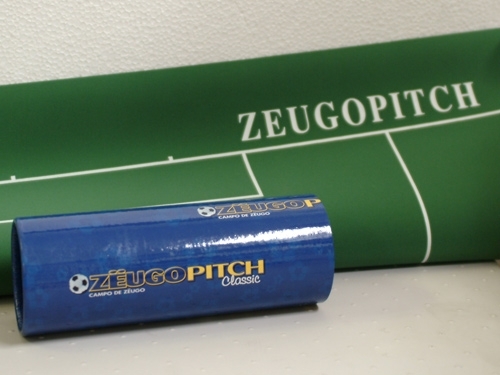The product image features a green mat, known as Zoogo Pitch, with white soccer field lines including the goal box and goal area, making it suitable for tabletop play. The mat has "Zoogo Pitch" written in white, with "Classic" in cursive underneath. Accompanying the mat is a dark blue, shiny tube case, which also bears the "Zoogo Pitch" inscription in yellow letters and a blue outline around "Zoogo". The tube features a distinctive logo with a soccer ball next to the 'Z'. The entire setup is displayed against a light gray or beige background with a subtle pebbling texture visible at the top. The right side of the tube showcases a noticeable bright white highlight, indicating its glossy surface.